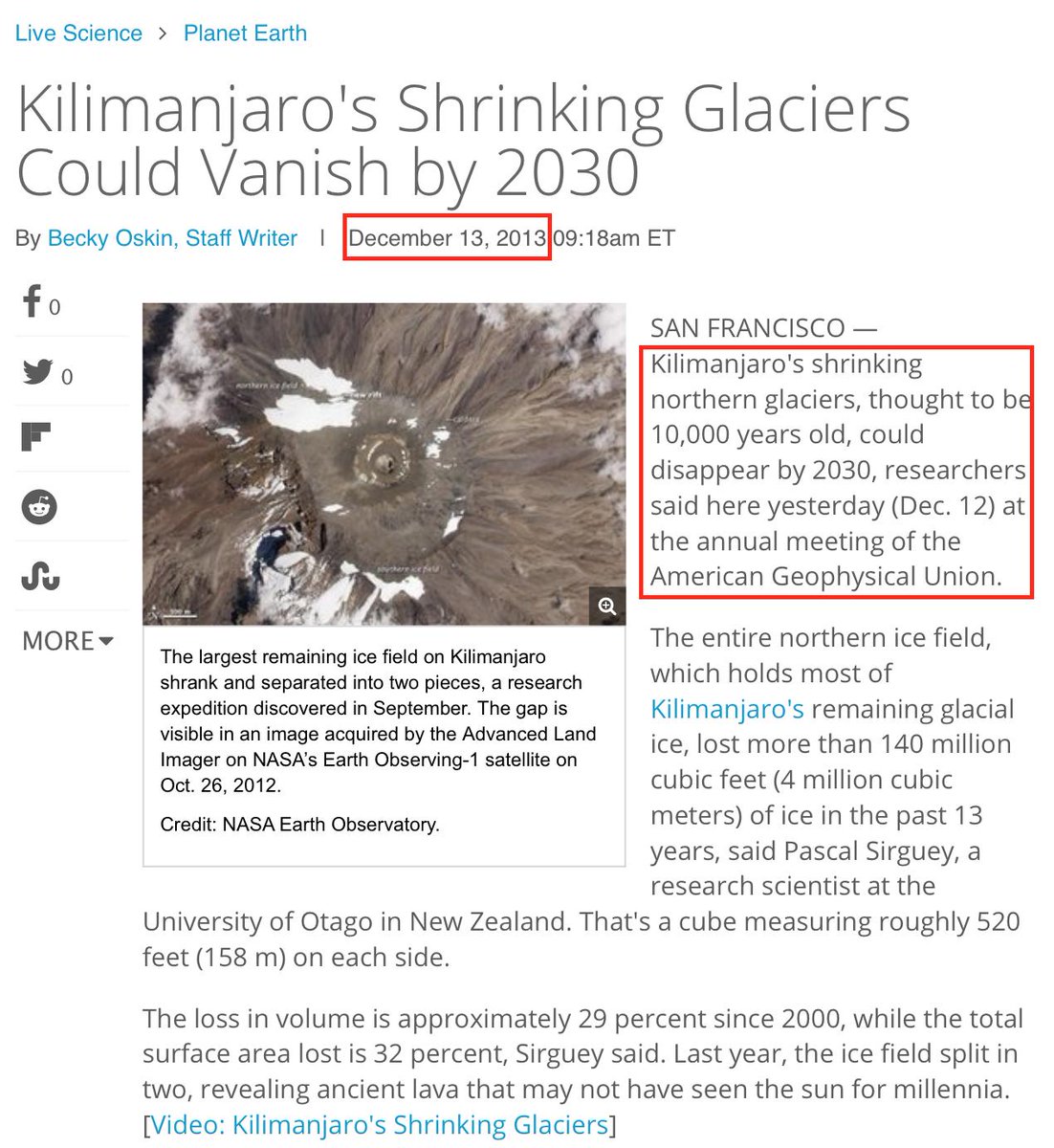Screenshot of a news article from LiveScience in the Planet Earth subcategory. The article, titled "Kilimanjaro's Shrinking Glaciers Could Vanish by 2030," is written by staff writer Becky Oskin. The publication date is December 13, 2013, at 9:18 AM Eastern Time, with the date highlighted and outlined in red. On the left of the article are social media icons for Facebook, Twitter, and Reddit.

The article includes an aerial photograph of Kilimanjaro's largest remaining ice field, which has notably decreased in size and split into two pieces. This significant change was documented by a research expedition in September and captured by NASA's Earth Observing 1 satellite on October 26, 2012, via the Advanced Land Imager. The photograph, credited to NASA Earth Observatory, predominantly shows a brown crater with minimal white ice patches.